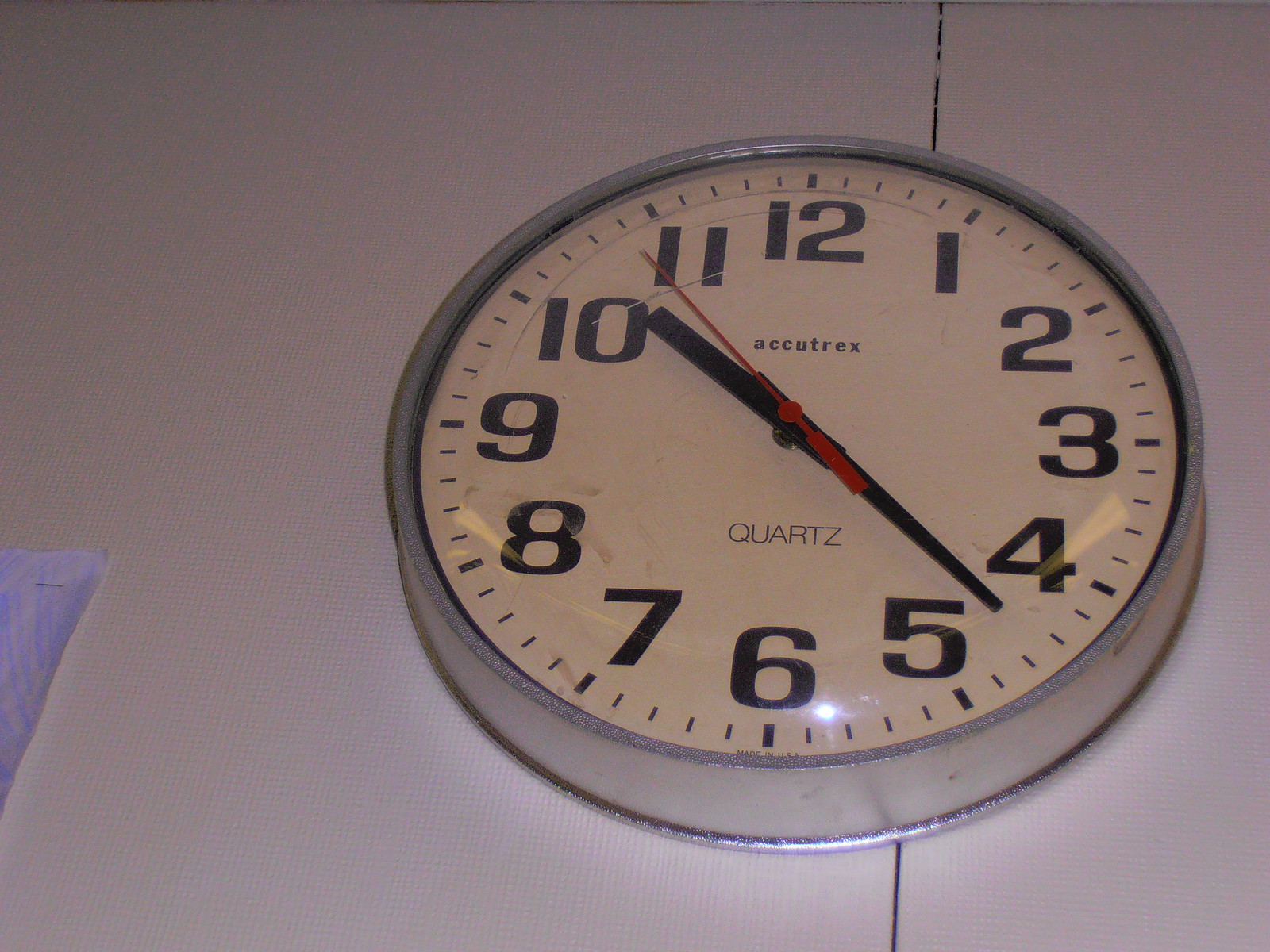This image features a standard wall clock that would commonly be found in a government office or business setting. The clock is mounted on a gray wall, which appears to be made up of partition panels often used to create cubicles in office environments. The clock, branded Accutrex, has a chrome metal frame with a classic off-white face displaying large, bold black numbers. The minute and hour hands are black, while the second hand is red. The time displayed is 10:22, close to 10:23. In the background, a piece of paper, likely a child's drawing with blue crayon, is stapled to the wall panel below the clock. Additionally, the clock face features a small crack in the upper left section of the glass. The clock indicates 'quartz' at the bottom of its face and has fine lines marking the minutes between the bold numbers.